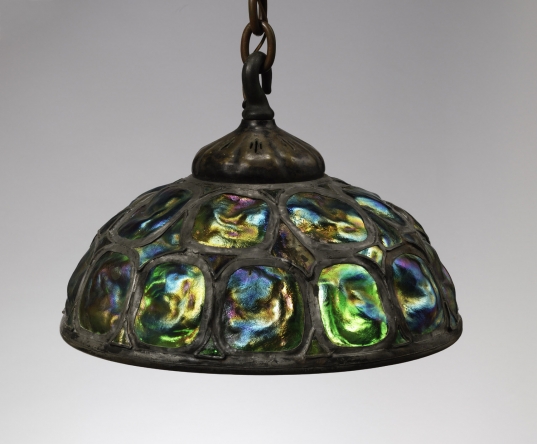This photograph features a rustic, handmade hanging lamp suspended by a chain and hook, designed to illuminate a space such as a dining table. Crafted in an artistic style reminiscent of a more rudimentary Tiffany creation, the lampshade is composed of round disks of colored glass joined together by thick, black solder. The multicolored glass varies in shades of blue, green, brown, gray, and white, giving it a stained glass appearance. The fixture has a circular design and multiple layers of glass that create a unique play of light depending on the angle of illumination. The intricate yet simple craftsmanship, devoid of any mass-manufactured elements or additional accessories, gives this one-of-a-kind piece its distinctive, rustic charm. The background of the image is plain, focusing solely on the lamp in the center.